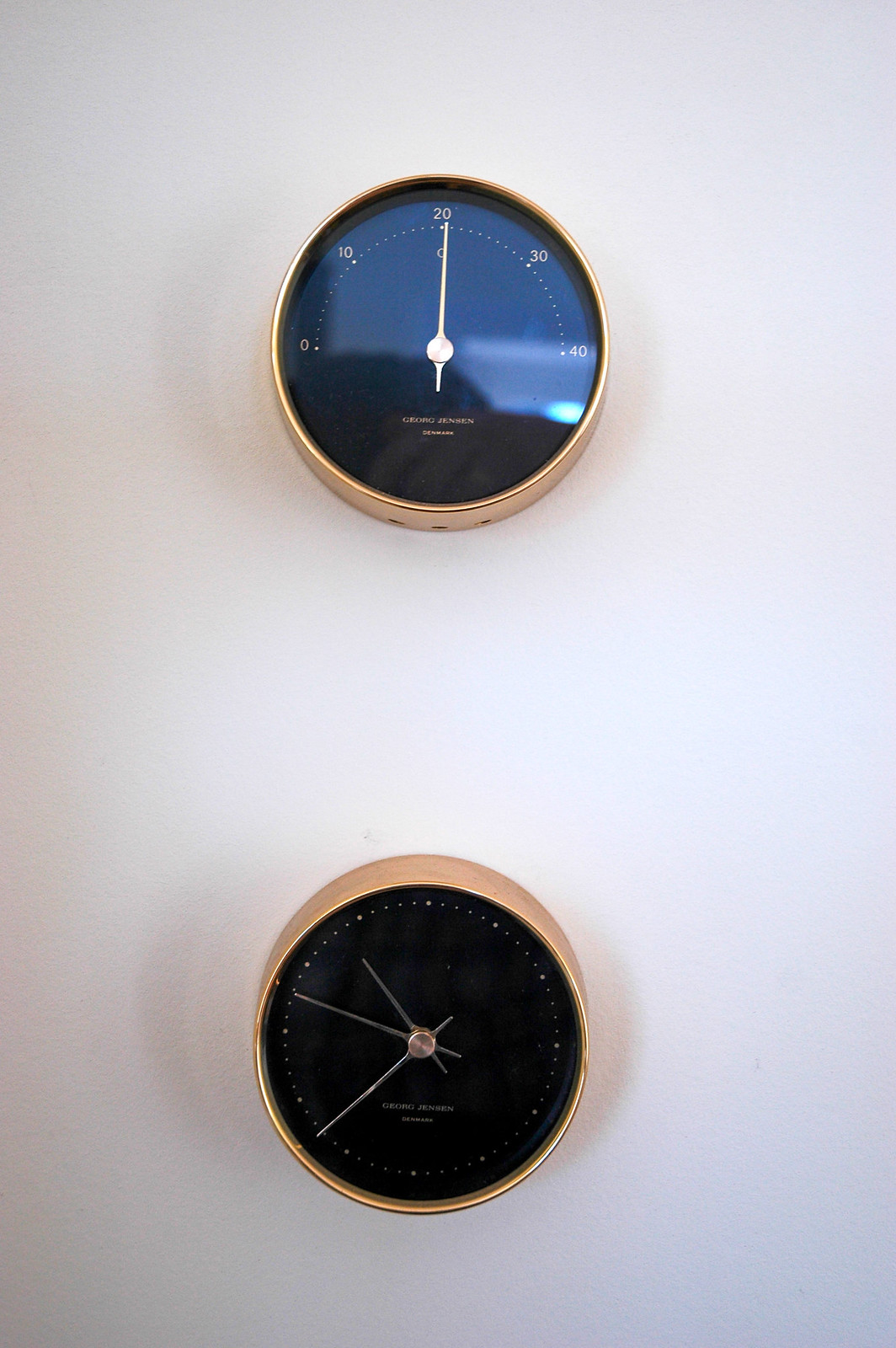This image displays two circular brass-framed devices mounted on a pristine white wall. The upper device, which resembles a clock but is actually a barometer, features a black face with elegant gold lettering that reads "Georg Jensen." Its brass needle points to the 20 mark, situated in the middle of the scale, suggesting atmospheric pressure readings denoted by numbers 0, 10, 20, 30, and 40 arranged in an arc.

The lower device is an actual clock, sharing a similar design aesthetic with a black face, brass outer ring, and gold lettering that also reads "Georg Jensen." This clock has brass hands pointing to the time 10:40:50. The clock face is marked with large dots representing the hours from 1 to 12, while smaller dots are placed between each hour mark to denote 15-minute intervals, contributing to both its functionality and visual appeal.